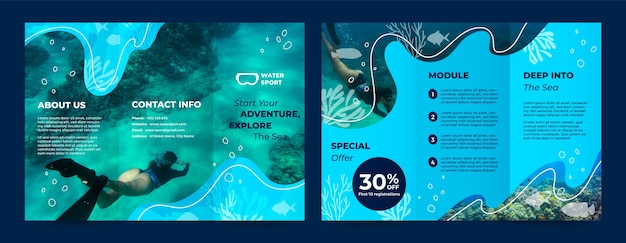The image features a detailed, aquatic-themed advertisement brochure laid out flat, revealing both the front and back panels. The brochure is designed with creases for a trifold format. It has a dark blue frame and an underwater background, split into two main sections, depicting scenes of ocean exploration. 

On the left side, there is a vivid underwater photo showing a diver with flippers, swimming among digital art illustrations of underwater plants and fish. The headings on this side include "About Us" and "Contact Information". Another key heading here states “Start Your Adventure, Explore the Sea,” accompanied by an image of goggles labeled “Water Sport.”

The right side of the brochure continues the underwater theme, presenting fish in the corners and coral at the bottom. Prominently featured is a large black circle with white text that reads “30% Off,” indicating a special offer. This section also includes the headings “Module” with four paragraphs of indecipherable small text beneath it, and “Deep into the Sea.”

The unified depiction and repeated elements across both panels create an inviting, adventurous theme, encouraging viewers to engage with underwater activities and explore the sea.